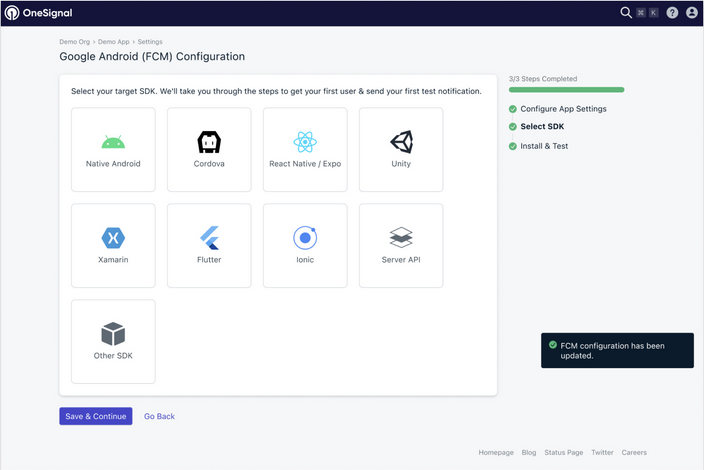This screenshot captures a specific window from the OneSignal software application, meticulously cropped to exclude any extraneous desktop details. The open window prominently displays the title "Google Android (FCM) Configuration," indicating it is part of a setup process for configuring communication between platforms using Firebase Cloud Messaging. Within this window, users can select a target SDK from a series of square, logo-embellished boxes. Each box represents a different platform or development framework, including options like Native Android, Cordova, React Native, Unity, Xamarin, Flutter, Ionic, Server API, and Other SDK. Choosing one of these selectable targets guides the user through a series of steps to set up notifications, ensuring a seamless integration process for developers working with varied technologies.